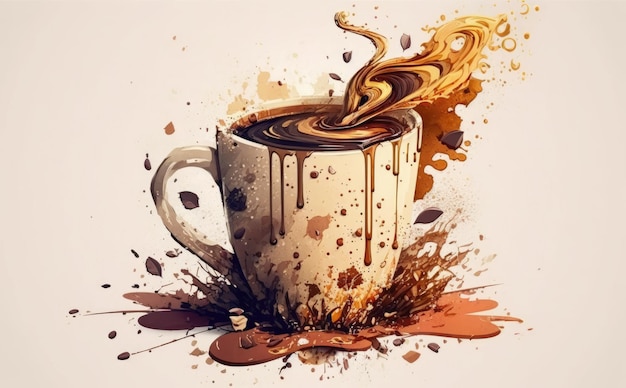The image is a detailed, artistic rendering, possibly a cartoon, CGI, or painting, featuring a central white coffee mug filled with dark brown coffee. The background is a tannish white color, contributing to the overall cohesion and simplicity of the setting. Emerging from the cup is a vivid, chaotic explosion of liquid in various shades of brown, beige, and tan, giving the impression that something has been dramatically thrown into the coffee. This splash effect extends in dynamic swirls and splatters around the cup, with drips cascading down its sides. The base of the image depicts the mug placed in a large, impactful paint splatter, further contributing to the sense of motion and chaos, as if the cup has been forcefully slammed into the puddle beneath. This amalgamation of lively splashes and drips creates an overall impression of energetic disarray while maintaining an artistic quality.